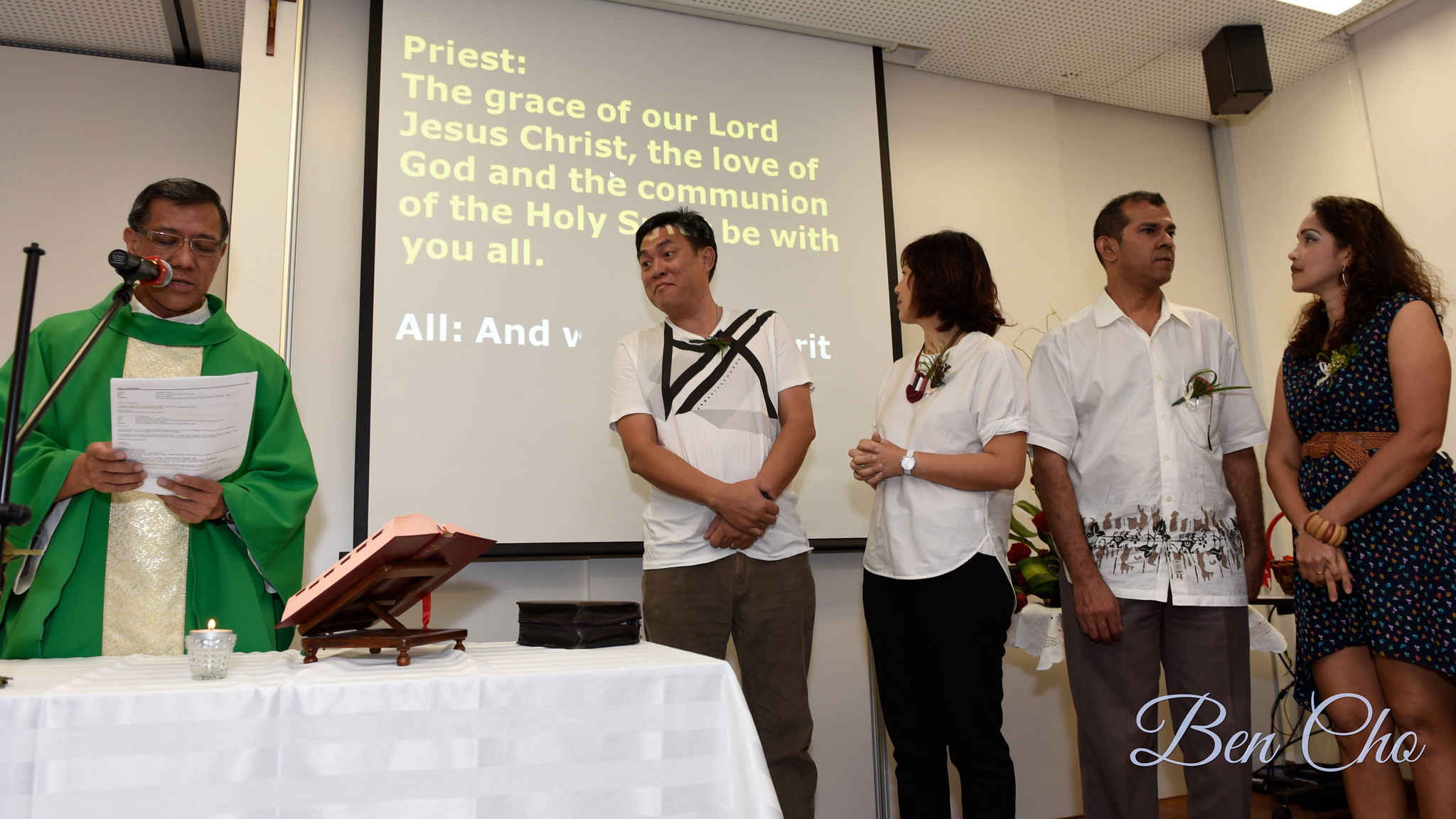In this image captured at a church function, we see five individuals positioned in front of a white wall with a projector screen pulled down. The screen displays a spiritual message: "Priest: The grace of our Lord Jesus Christ, the love of God, and the communion of the Holy Spirit be with you all." The text is in white letters set against a grey background. On the left side of the image stands a priest, identifiable by his green robe. He is speaking into a microphone mounted on a metal pole, while holding a piece of paper. In front of him, a table draped with a white tablecloth displays an open book and a lit candle, indicating a formal setting. 

To the right of the priest, four people are standing. The first man, closest to the priest, is dressed in a white top and brown pants. Next to him is a woman wearing a white top and black pants, her black hair flowing as she looks back at the screen. The next man in line sports a white shirt with embroidery at the bottom and grey pants. The final woman in the group is dressed in a black skirt with polka dots, just above her knees, and her long black hair cascades down as she also gazes toward the screen. On the bottom right corner of the photo, the name Ben Cho, written in cursive, adds a personal touch to the image.